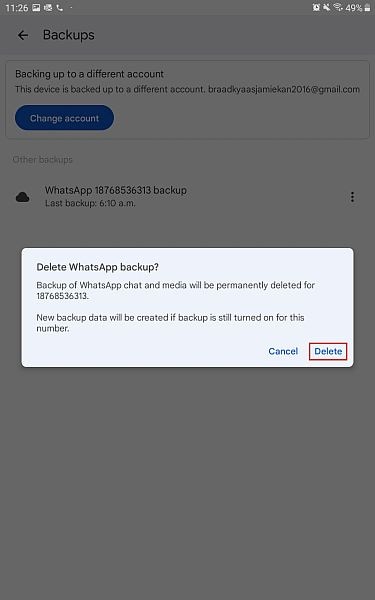The image features a grey background with a smartphone interface at the top. On the top left, white text reads "1126" inside a white square indicating the time. To the right, there are additional icons including a clock, Wi-Fi signal, and battery life, which is at 49%.

Below this, on the left side, there's a black arrow pointing left with the word "backups" in black font on the grey background, followed by a grey line underneath. Under this section, on a white background with black text, it states: "backing up to a different account." It further explains that the device is backed up to a different account and offers an option to "change account," presented in white font within a blue circle.

Just below, grey text reads "other backups," followed by a section involving a black cloud icon. Next to it, in black font, it says "WhatsApp," and a number "187-685-36313," indicating a backup. Beneath, it mentions the "last backup" was at "610 AM," with three dots to the right in a white square with black font, providing a menu option.

The subsequent text explains: "delete WhatsApp backup?" and asks whether the backup of WhatsApp chat and media will be permanently deleted for the contact "187-685-36313." It further notes that "new backup data will be created if backup is turned on for this number."

On the right, there are options with "cancel" in blue text, and beside it, "delete" in red text with a red border, giving a choice to proceed with the action or not.